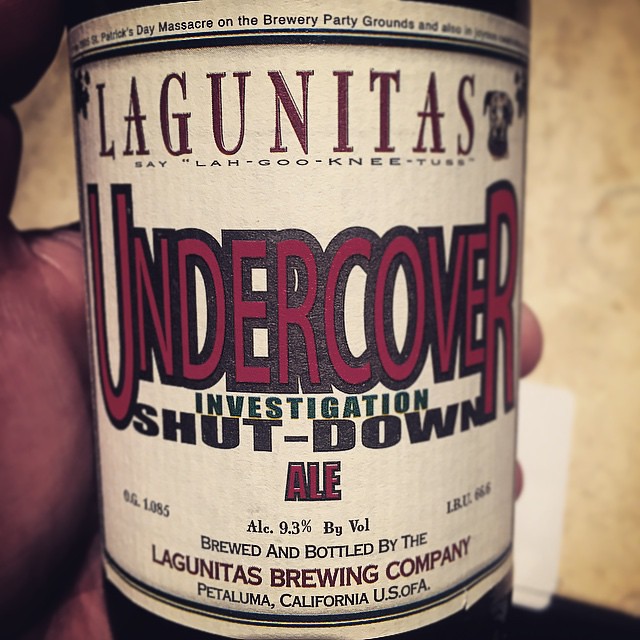This full-color photograph captures a close-up view of a beer label being held up to the camera by a hand. The label features a light tan background with red and black text prominently displaying "Lagunitas" at the top. Below it, the beer's name reads "Undercover Investigation Shutdown Ale" with an alcohol content of 9.3% by volume. The text also assures the correct pronunciation of "Lagunitas" with a phonetic guide: "say La-gu-ni-tas." This ale is brewed and bottled by the Lagunitas Brewing Company, headquartered in Petaluma, California, USA. The label also alludes to an event called the "St. Patrick's Day Massacre on the Brewery Party Grounds," drawing a comparison to the infamous St. Valentine's Day Massacre. Additional details, such as the term "OG1085," are visible but obscure in meaning. The label's text is set in aesthetically pleasing burgundy and black fonts, adding to its visual appeal on what is clearly identified as a glass bottle.